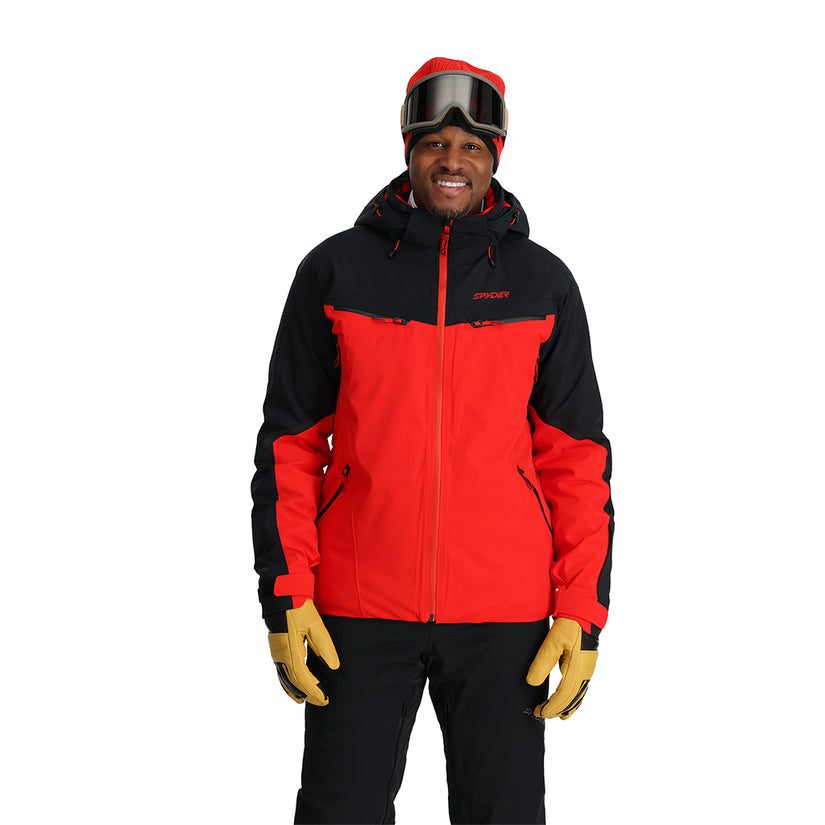This image features an African-American man in his 30s or 40s, smiling and looking directly into the camera. He has a short beard and mustache and is wearing a red knitted cap with black detailing at the bottom. On his forehead rests a pair of black and gray ski goggles. He is dressed in a winter jacket that is predominantly red with black sections along the collar, shoulders, and the outer parts of the arms. The jacket has a red logo on the right breast that reads "SPYDER." He is also wearing black pants and thick yellow gloves with black accents. The photo is taken against a plain white background, and the man is posing with his hands at his sides, appearing to model the winter gear.